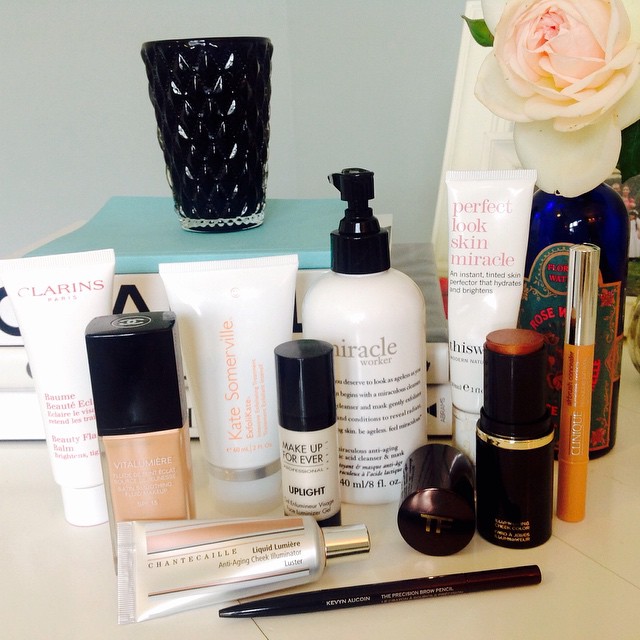On a pristine white tiled vanity countertop, a neatly arranged collection of beauty products is displayed. From left to right, the lineup begins with a container from Clarins, distinguished by its light red lettering on a white background. Adjacent to the Clarins product is a tube of liquid foundation makeup. Following this is a series of tubes from the renowned skincare brand Kate Somerville. A small black and white tube labeled "Make Up For Ever," which appears to be a cosmetic product rather than lipstick, is next in line.

A white container with a sleek black spray pump, inscribed with the words "Miracle Worker," occupies a central position among the items. In the foreground, there is a dark pencil-like object, resembling either an eyebrow pencil or an eyeliner, adding to the assortment of makeup tools. To the far right, a tube of Clinique mascara is visible. Adding a delicate touch to the scene, a pale pink and white rose is positioned in the upper right corner amidst an array of other bottles, completing this meticulous display of beauty essentials.